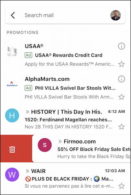This image appears to be a low-resolution screenshot from a mobile device, possibly a smartphone or a tablet. At the top of the screen, the "Search mail" bar is prominently displayed. Next to it, there's a circular icon featuring a blurry picture of a man, though the details of the image are indistinguishable. Below the search bar, several email listings are visible, but the text is largely unreadable due to the resolution. However, some recognizable elements include a label that seems to read "Promotions" and email senders such as USAA, Alphamarts.com, and history-related content from "This Day in History."

One particular email is highlighted, and a red section with a trash can icon is visible on the left side, suggesting an option to delete this email. The email appears to be from a sender with a partially readable email address ending in ".com." Additionally, another listed email includes a "W" icon and a subject line mentioning "W-A-I-R" and "Plus Deep Black Friday."

Overall, this screenshot captures someone's email inbox on a mobile device, emphasizing a highlighted email poised for potential deletion.